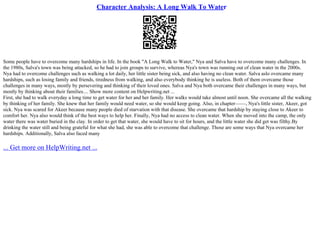The image appears to be a digital screenshot featuring a character analysis for a text titled "A Long Walk to Water," with the headline written in blue letters. Below the headline, there is a black QR code consisting of a large black square with three smaller squares in the top-left, top-right, and bottom-left corners, resembling the static of an old black and white television. The QR code is intended to be scanned with a smartphone for more information. Beneath the QR code, there is a passage of text that is very small and illegible without a magnifying glass. At the bottom of the image, also in blue writing, it says "get more on helpwriting.net," flanked by three blue dots on each side and a blue underline. The purpose of this image is unclear without further details provided by the QR code.